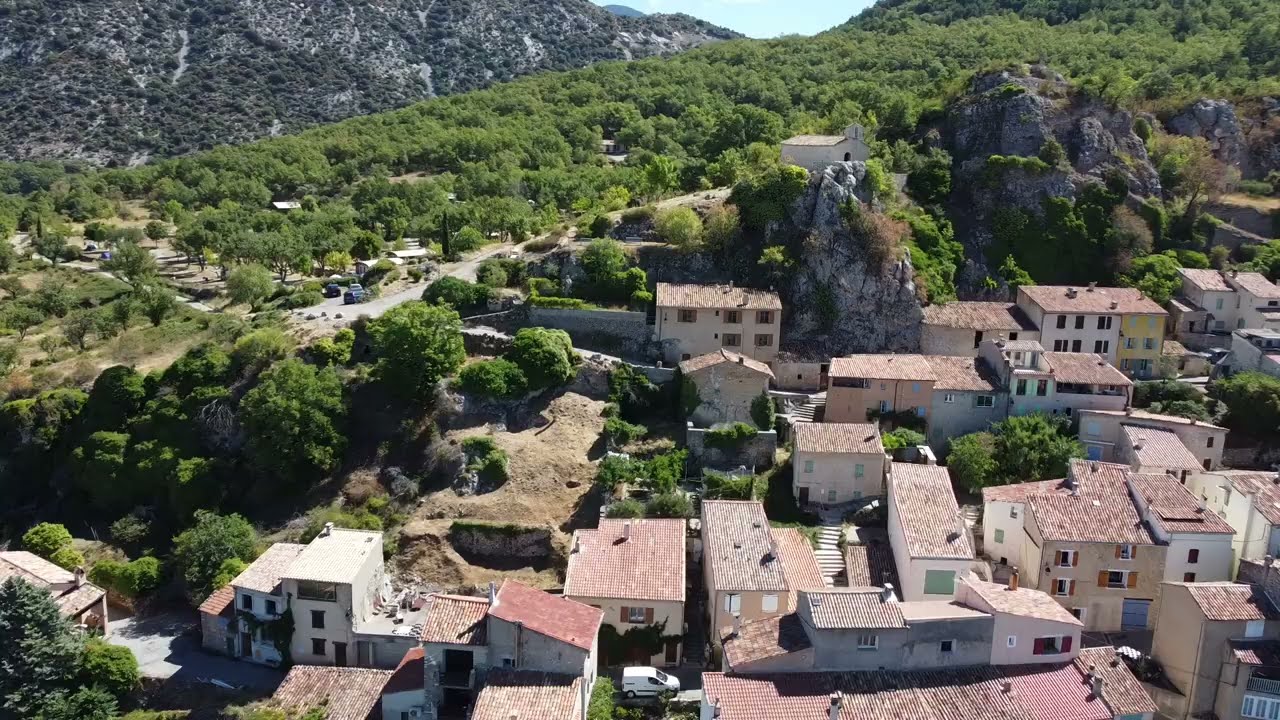The image is a photorealistic aerial view of a small town nestled in a hilly, rocky region on a bright sunny day. The town occupies the bottom half of the image and consists of numerous buildings with roofs predominantly in neutral tones of brown, light blue, and gray, often reddish or orange-hued. These structures, likely residential, suggest a quaint, possibly European or Southwestern U.S. aesthetic. Towards the top right, imposing gray stone cliffs are adorned with pockets of greenery. In the top left area, a dense patch of vibrant green trees partially obscures some of the buildings, providing a lush contrast to the more barren rocky hills behind. Further up and to the left of the image, a larger, darker green hillside ascends, culminating in a rocky mountain that dominates the backdrop. A clear blue sky stretches across the top center, framing the tranquil yet varied landscape captured in this stunning overhead shot.